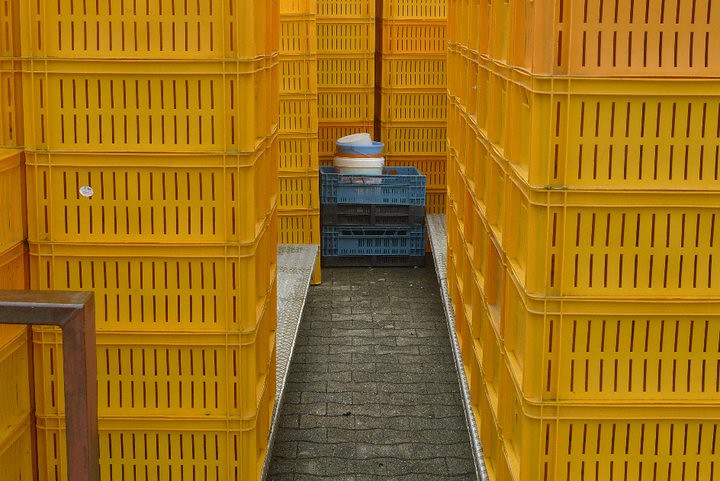The image depicts a scene that appears to be at or outside a warehouse, with numerous plastic fruit boxes prominently featured. To the right, left, and back, there are stacks of yellow plastic crates with slits on their sides, likely designed for transporting items that need ventilation, such as fruits or vegetables. These yellow crates are stacked on top of steel platforms with red metal lines around them, possibly for stability or safety during handling.

In the center of the image, there are two blue crates and two black crates, neatly piled on top of each other. These central crates contain four buckets—two white, one brown, and one light blue. One of the blue crates at the top visibly holds these buckets. The scene's composition leads the viewer's perspective from the bottom to the middle, drawing attention to the different colored crates.

The entire arrangement is set on a gray brick or cobblestone surface, adding to the industrial atmosphere of the warehouse.